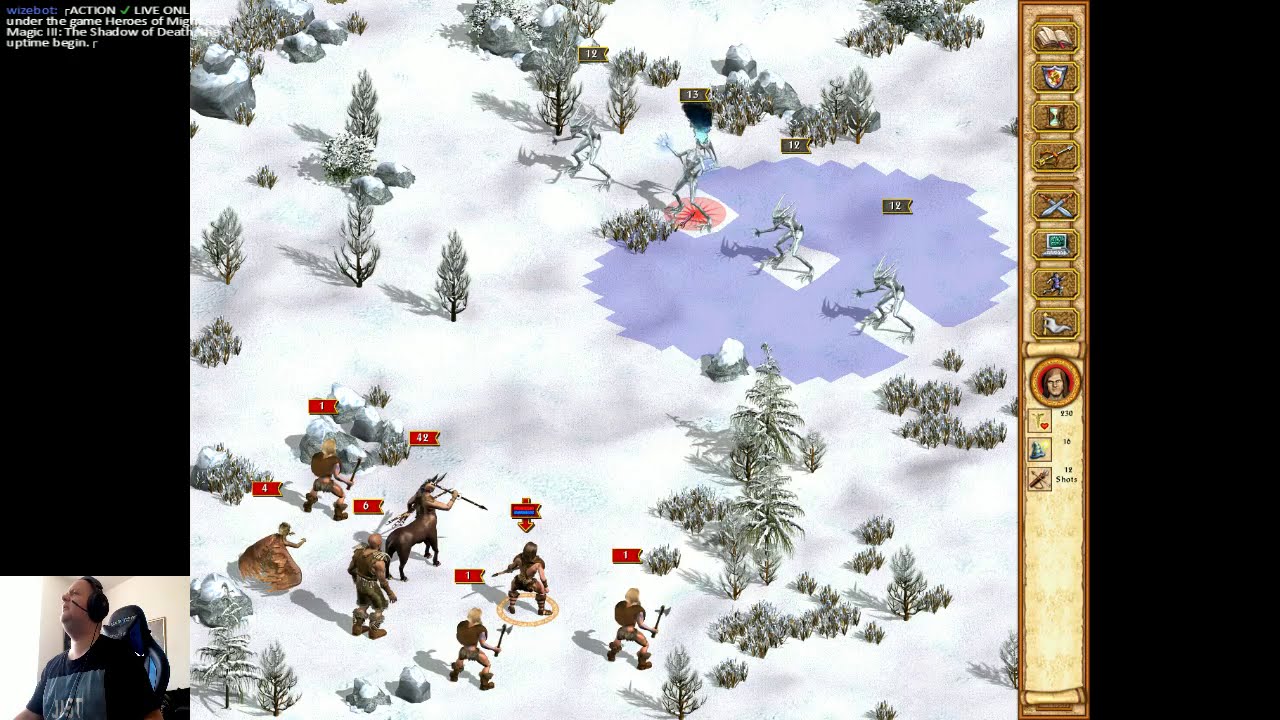This image is a detailed screenshot of a live stream where a gamer is playing a real-time strategy (RTS) game. In the bottom left corner, we see the player through a webcam, sitting in a black gaming chair and wearing a black t-shirt with a logo, along with a black headset that has a microphone. Behind the gamer is a plain white wall, suggesting he is in a simple indoor setting.

The main focus of the screenshot is the game itself. The game presents a snow-covered terrain dotted with pine trees and small shrubs, with icy patches evident on the landscape. There is a medieval warrior theme, featuring a diverse army of characters including warriors in brown attire wielding battle axes and spears, a Cyclops, and a centaur brandishing a spear. These forces appear to be preparing for battle against enemy creatures resembling skinny, silver-colored gargoyles, skeletons, and zombies positioned on a frozen pond.

The game interface includes several elements: on the far right, there is a vertical inventory bar showcasing various items within a brown rectangular frame, and on the upper left, a chat window is barely visible. Distinctive visual aids like colored banners with numbers above characters help differentiate factions, with red banners and yellow numbers for one side, and gray and white for the opposing side. This caption encapsulates the detailed and dynamic environment captured in the live-streamed gameplay screenshot.